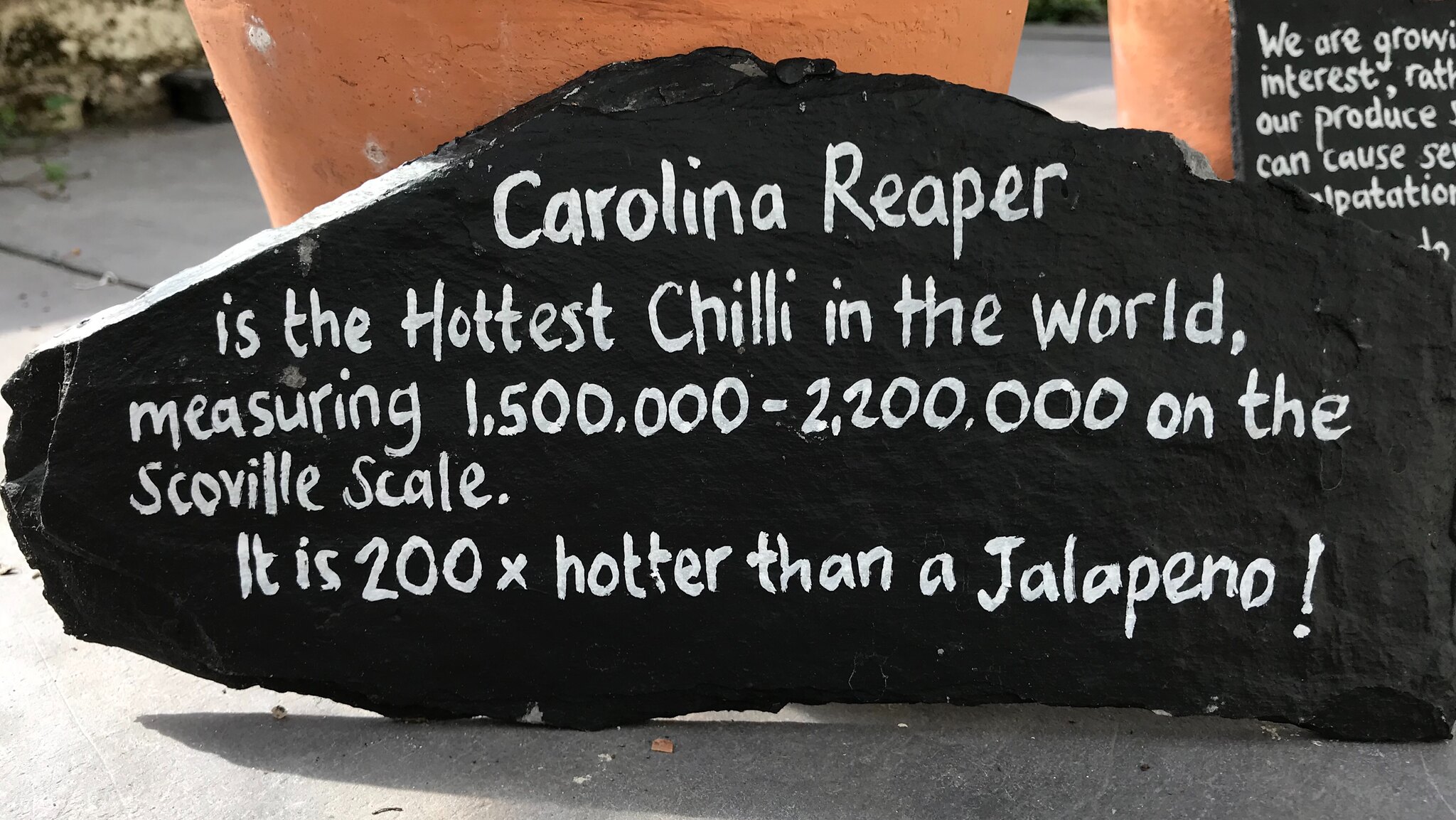The image displays a close-up of a large, black-painted stone sign, centrally positioned on gray asphalt in an outdoor market setting. Handwritten in white paint, the sign declares, "Carolina Reaper is the hottest chili in the world, measuring 1.5 million to 2.2 million on the Scoville scale. It is 200 times hotter than a jalapeno." In the background, there are potted plants and another black stone sign with partially legible white text. The composition suggests an informative display about Carolina Reaper chilies, likely at a farmer's market.